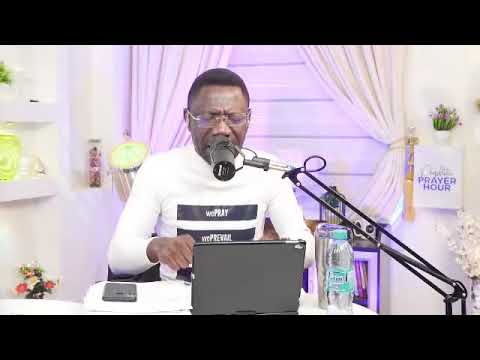In the image, a dark-skinned African American man is the focal point, meticulously positioned at the center of the photograph. The setting appears to be indoors with a warm and organized arrangement typical of a live stream or podcast environment. He is seated at a table with several items in front of him: a laptop, a cell phone to his right, a silver water bottle, and a microphone held close to his mouth, indicating he might be speaking or singing. He is dressed in a long-sleeved white turtleneck shirt adorned with black horizontal lines featuring the text "We Pray and VTC Prevail," although the details of the text are a bit blurred.

Enhancing the composition, the background features white walls with white shelves to the left, showcasing various ornaments. To the right of the man, there is a decoration with the text "Prayer Hour" in purple font, and a white pot with green stems and small purple flowers sits atop it. Additional elements include a window framed by curtains, contributing to the cozy ambiance. A light lavender purple glow illuminates the scene from behind, adding a serene touch to the photograph's color palette, which includes shades of white, green, light green, pink, black, gray, purple, and light blue. Overall, the photograph captures a detailed moment of focused engagement within a well-arranged and purposeful indoor setting.